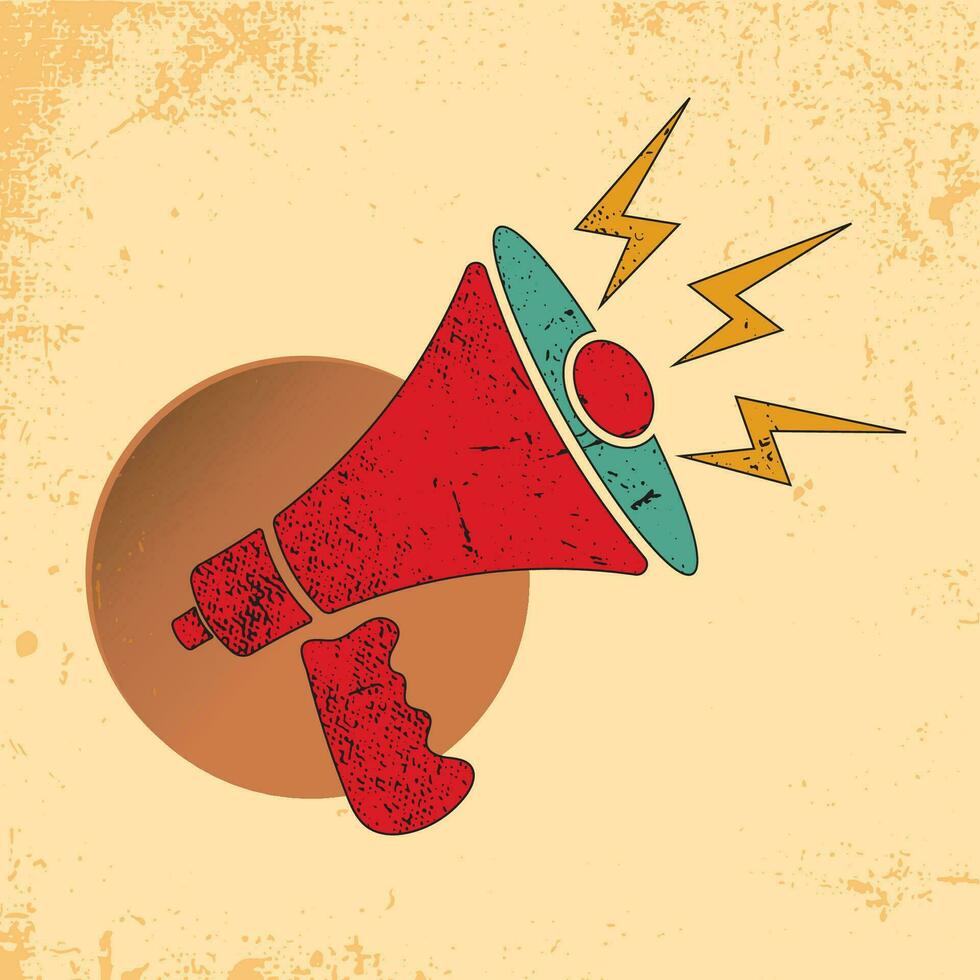This vertically rectangular image features an artistic rendering of a red megaphone set against a light yellow-brown or beige background with sporadic darker spots on the top left and right corners. The lower left of the background showcases a dark, brownish-orange circle that anchors the base of the megaphone. The megaphone itself, facing right, has a detached handle and segmented parts, with a turquoise interior and a red ring at its center. Extending from the megaphone's bell are three jagged yellow lightning bolts that symbolize sound waves. The composition suggests an illustration or painting, possibly with a small signature in the bottom right corner.